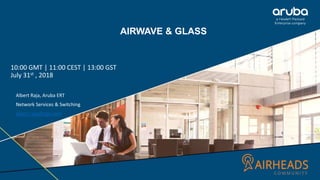The image titled "Air Waving Glass" features a detailed and visually rich advertisement. In the top right corner, the name "ARUBA" is prominently displayed. Just below the title, on the left side, the advertisement lists three times: 10 GMT, 1100 CEST, and 1100 GST, along with the date July 11, 2018. These elements are set against a striking blue triangular background.

Below this blue triangle, the image transitions to depict the inside of a building lobby. Here, a man and a woman are seen seated together. The man, positioned on the left, is dressed in a white t-shirt and black tie, with a laptop on his lap. The woman sits to his left, intently gazing at the laptop screen. This scene appears somewhat blurry, adding a soft focus effect to the overall image.

In the bottom right corner of the image, the word "Arrowheads" is displayed. There's also a mention of the text "Airheads" in orange, positioned next to a drawing of a radio tower, which adds a unique graphical element to the advertisement. The layout and details collectively create a visually engaging narrative.